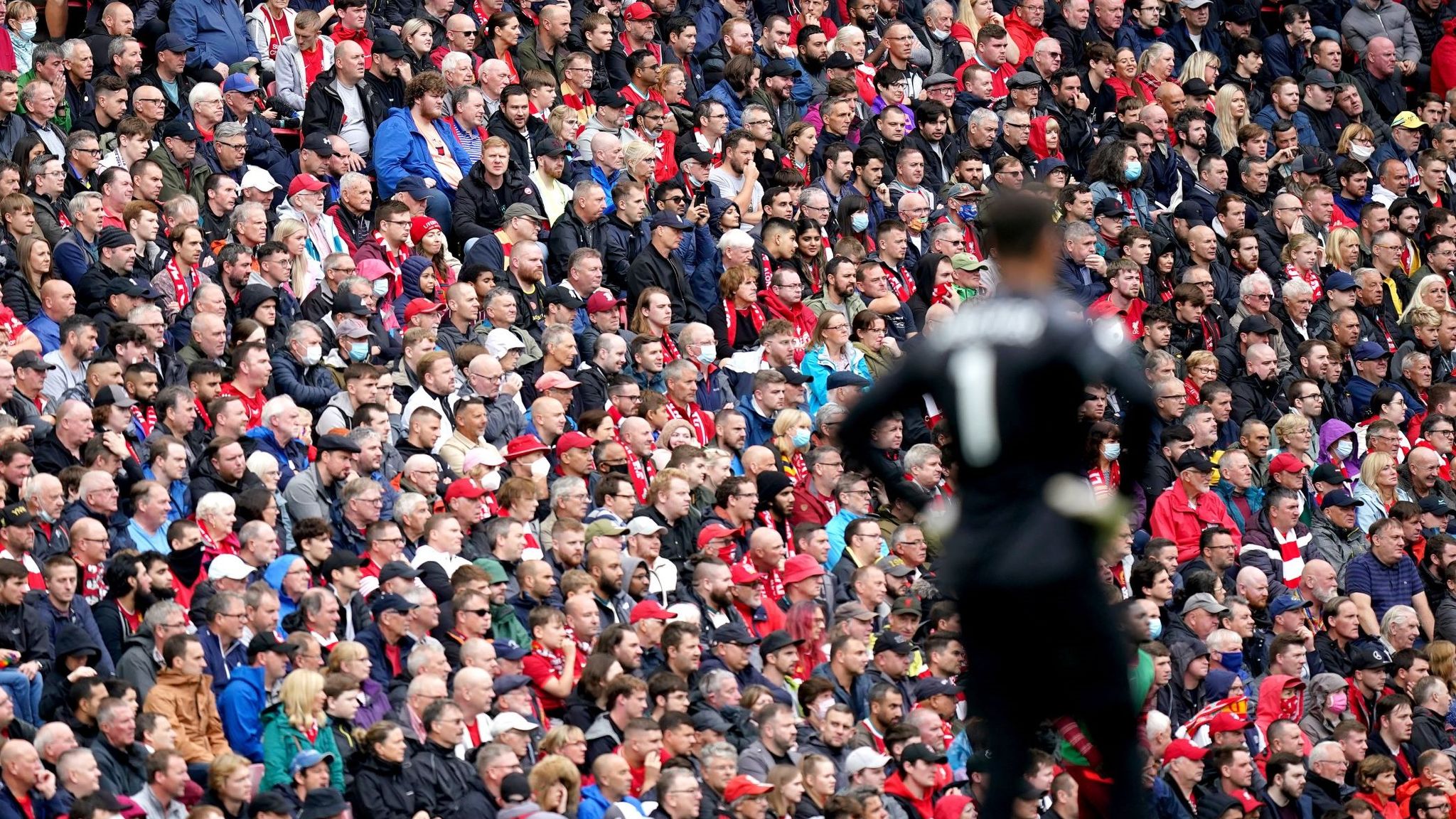The image captures a vibrant scene within a rectangular stadium, teeming with a massive crowd of spectators. Rows upon rows of diverse faces—men and women of various ethnicities, though predominantly white—are focused intently towards the right side of the stadium. Most of the spectators are clad in an assortment of colors, notably a substantial number in red, presumably supporting their team, and many don hats and caps. The scene is set in daylight, enhancing the clarity and energy of the moment.

In the foreground, a soccer player with his hands on his hips stands prominently. He wears a black jersey and black shorts, with the number one visible on his back. His name is blurred, and his brown hair and white skin are distinguishable despite the blur. He appears to be deep in thought, perhaps a goalkeeper observing the game unfolding ahead of him, his gaze fixed towards the right where the eyes of the crowd are also directed.